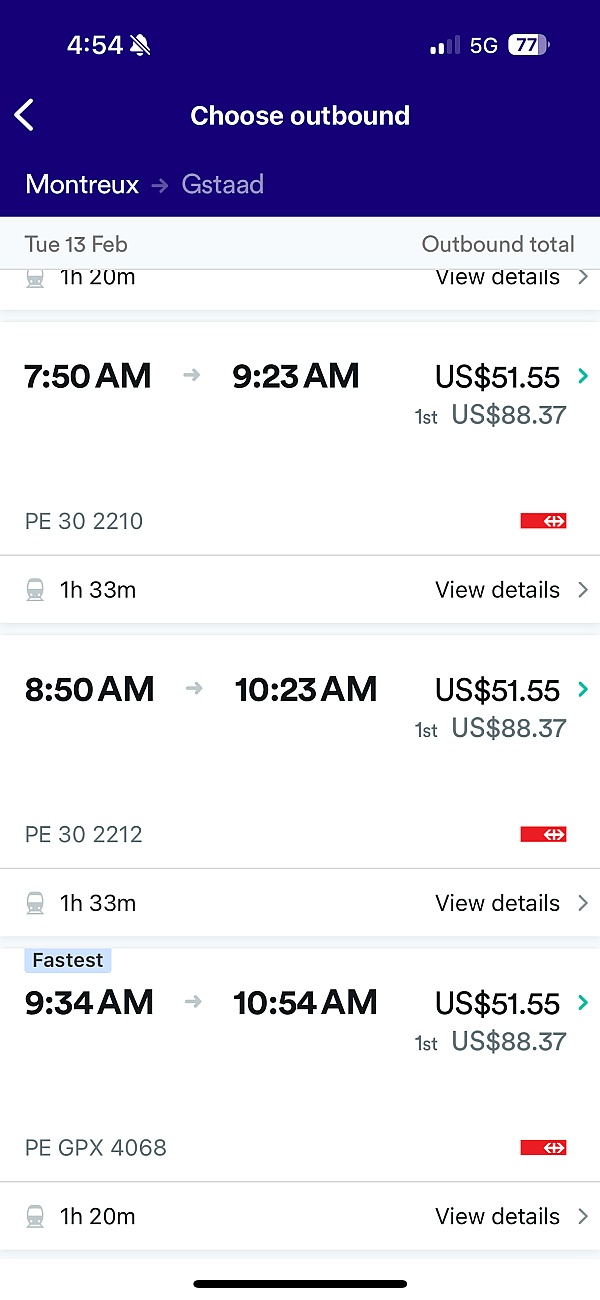In the screenshot, we observe a flight booking page displayed on a mobile device. The device time, shown at the top left, reads 4:54 AM, and the Do Not Disturb icon to its right indicates that notifications are disabled. On the top right, the network signal bar is at 2 out of 4 bars, accompanied by a 5G icon and a battery level of 77%.

The page is set for an outbound flight from Montreal, departing on Tuesday, February 13th. Three flight options are shown, all priced at $51.55. The first flight departs at 7:50 AM and arrives at 9:23 AM, with a total duration of 1 hour and 33 minutes. The second flight leaves at 8:50 AM and lands at 10:23 AM, also with a travel time of 1 hour and 33 minutes. The third and fastest flight takes off at 9:34 AM and touches down at 10:54 AM, consistent with the same duration of 1 hour and 33 minutes.